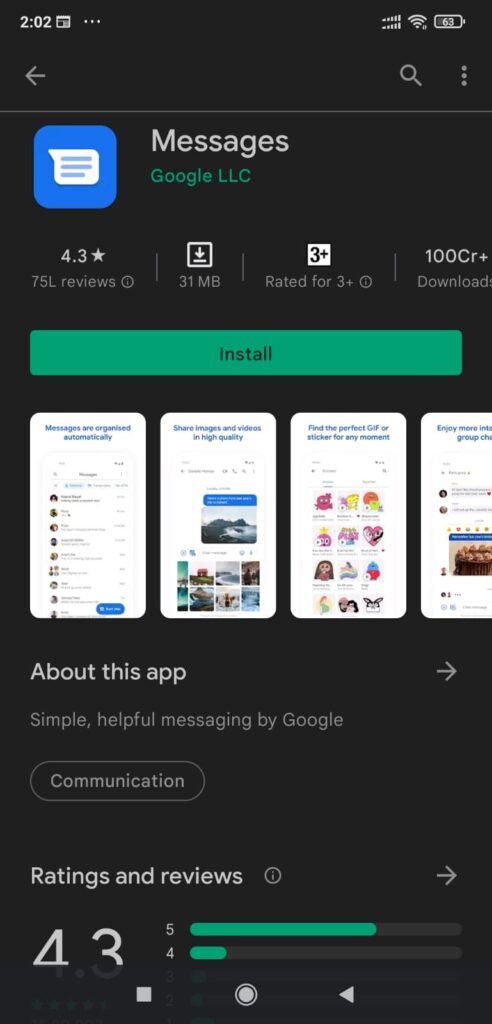The image depicts a smartphone screen displaying the Google Play Store page for the "Messages" app by Google LLC. At the top of the screen, the time is shown as 2:02, accompanied by a calendar icon, Wi-Fi signal indicator, and battery percentage icon. A white back arrow, magnifying glass (search icon), and a button with three vertical dots are also visible in the header.

Below the header, the app name "Messages" is displayed, followed by the developer "Google LLC" and the app icon—a blue background featuring a white speech bubble with blue lines inside. The app has a star rating of 4.3 based on 75K reviews. The download size is noted as 31 megabytes, and an arrow with a line beneath it indicates the download symbol. The app is rated for ages 3 and up and boasts over 100 million downloads. A prominent green "Install" button is available for downloading the app.

The screen also displays promotional images of the app, showcasing its interface, which includes contact lists and the ability to send images and other media. The "About This App" section features a white arrow pointing forward, and a tagline that reads "Simple, Helpful Messaging by Google." There is also a section for "Communication," and the "Ratings and Reviews" section with another white arrow pointing forward. The star rating of 4.3 is broken down into categories, displaying the distribution of 5, 4, 3, 2, and 1-star reviews.